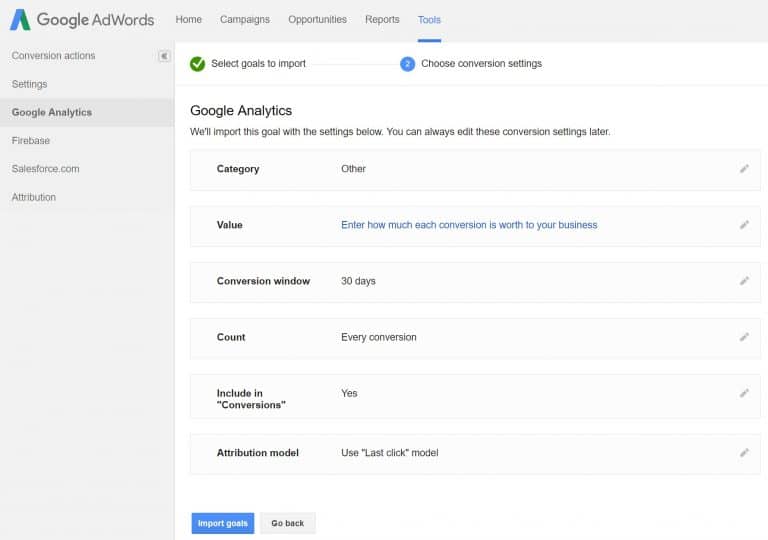This is a detailed screenshot of the Google AdWords website interface. At the top, there's a gray navigation bar. In the upper left corner, there is a logo consisting of an 'A' with a blue left side and a red right side, resembling an incomplete triangle. Adjacent to the logo, "Google AdWords" is written in a gray font.

To the right of the logo, there are several navigational selections: Home, Campaigns, Opportunities, Reports, and Tools. The "Tools" option is selected and highlighted in blue. Directly beneath the Google AdWords logo, there's a vertical menu on another gray bar with darker gray font. The menu items listed are Conversion Actions, Settings, Google Analytics (which is selected and highlighted in darker gray), Firebase, SalesForce.com, and Attribution.

To the right of this vertical menu, there is a prominent white main content window. At the top of this window, there's a green circle containing a white check mark, accompanied by the text "Select Goals to Import." A horizontal line extends to the right, leading to a blue circle with a white numeral '2', followed by the text "Choose Conversion Settings."

Beneath this, a black line separates the upper section from the lower section. The text below the line reads: "Google Analytics. We'll import this goal with the settings below. You can always edit these conversion settings later." Lastly, there is a gray rectangular box with the text "Category Other" written in black font.